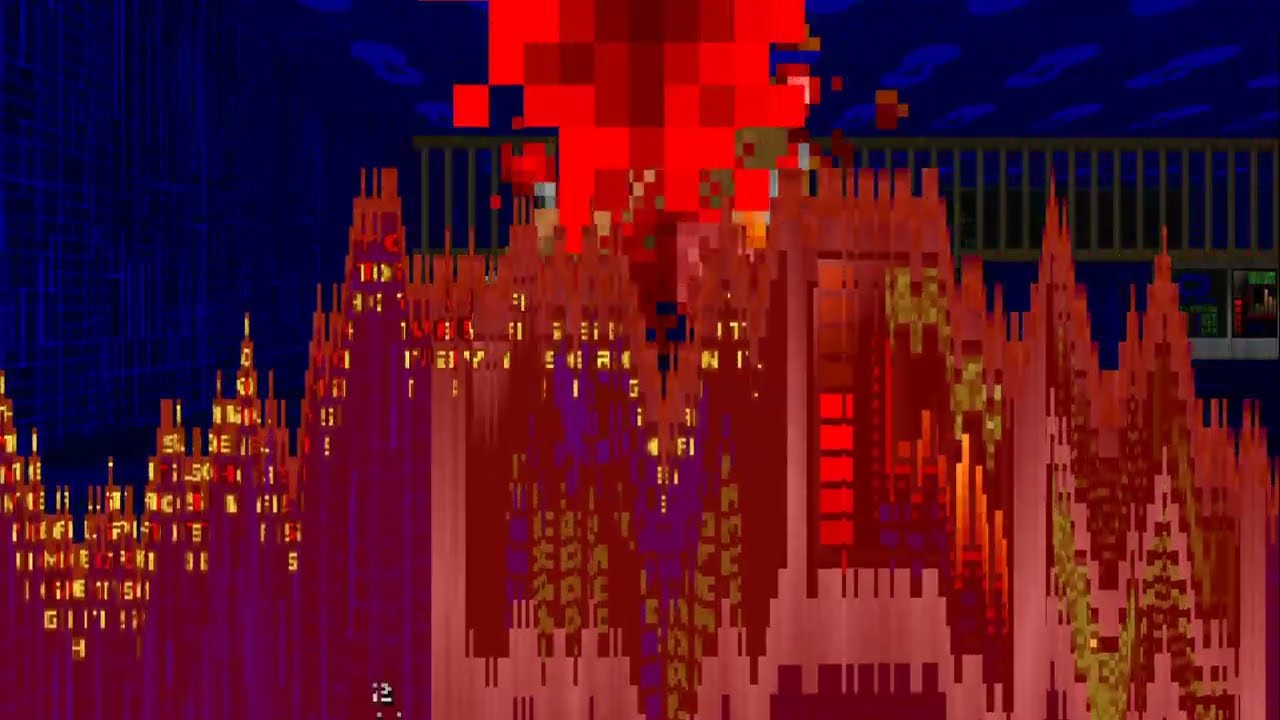This image appears to be a piece of intentionally pixelated digital art, resembling a glitching or crashing video game screen. Dominated by geometric shapes and a mosaic of colors, the scene includes what might be interpreted as purplish-pinkish mountains or buildings, topped with glowing yellow letters. The backdrop features a blue sky textured with intricate patterns that evoke computer circuits. In the center upper portion, there's a significant pixelated dark red blob.

Surrounding elements include a possible brown, fence-like structure and an ambiguous, blurry, black fence in the background. A white walkway is visible, coupled with a green sign on the right. The art conveys a sense of chaos and confusion through its severely pixelated, blocky aesthetic, with blue and black walls, light blue designs, and scattered yellow hues. Despite its abstract, three-dimensional ambience, the overall interpretation of the scene — whether it's depicting a crashing video game, a digitally-rendered landscape, or something else entirely — remains open to viewer interpretation.